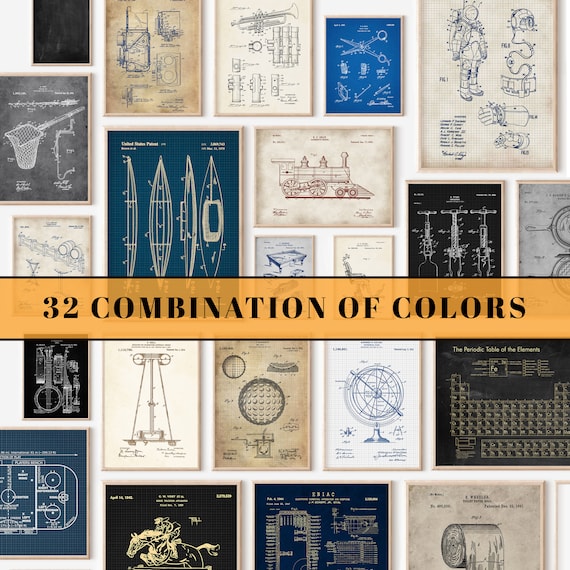The image displays a white wall adorned with a diverse assortment of framed prints, technical drawings, and sketches, covering a wide range of subjects from aircraft, motor vehicles, and mechanical diagrams, to boats, people, fishing nets, and even everyday objects like toilet paper and scissors. These framed pieces are not arranged in any particular order, spreading across the image without forming distinct rows, and are partially cut off at the edges. The prints feature a spectrum of colors, underlining the variety and detail in each design, with some images rendered in blue on a white background, others in white on a dark blue background, and some in black on beige. Dominating the center of the image is a yellow rectangular banner bordered in black, boldly proclaiming "32 combinations of colors" in black text, highlighting the diverse color palette available for these designs.